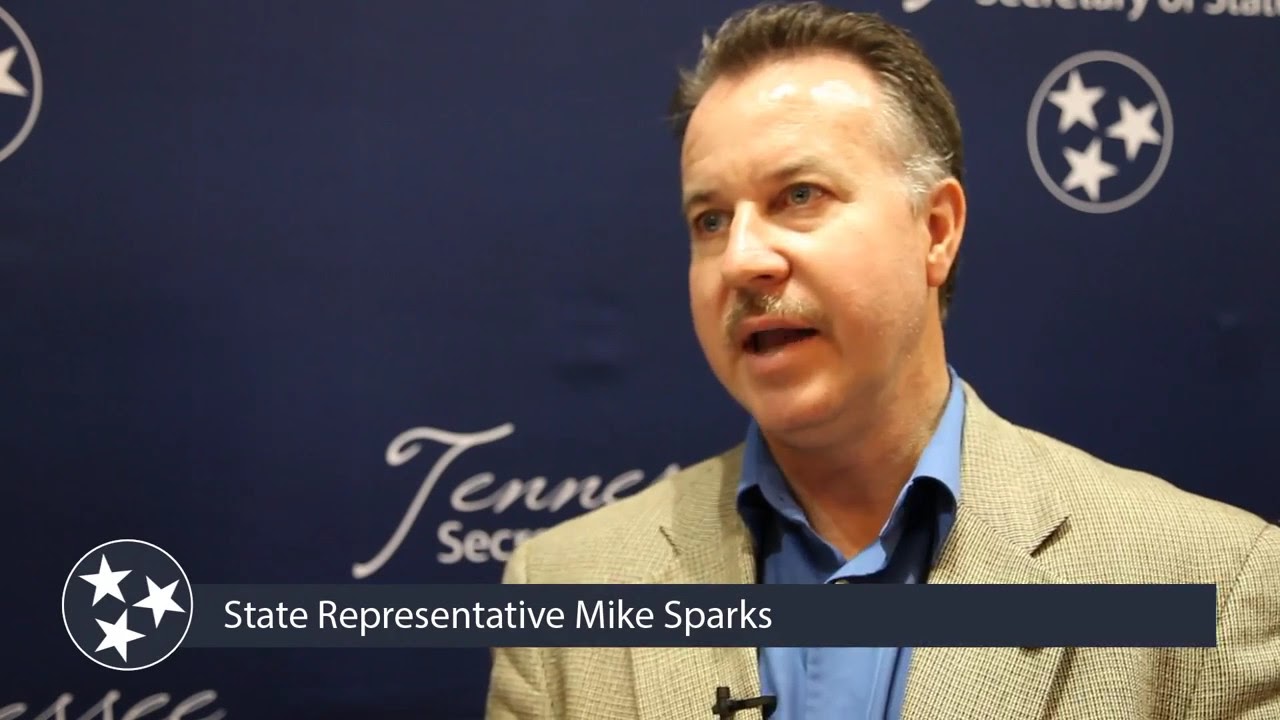The image is an advertisement or political campaign message featuring a white man identified as State Representative Mike Sparks. Standing towards the right side of the photograph, which is oriented horizontally, Sparks wears a tan blazer over a blue collared shirt and has a small brown and gray mustache. A microphone is visibly attached to his blazer, suggesting he is speaking, possibly in the context of a press conference or media gathering. The background is blue with a partial view of the word "Tennessee" and the top right features a logo of three white stars in a circle, partially mirrored on the left. A banner at the bottom bears the same three-star logo with the text "State Representative Mike Sparks." The colors in the image include black, white, beige, brown, gray, and blue.